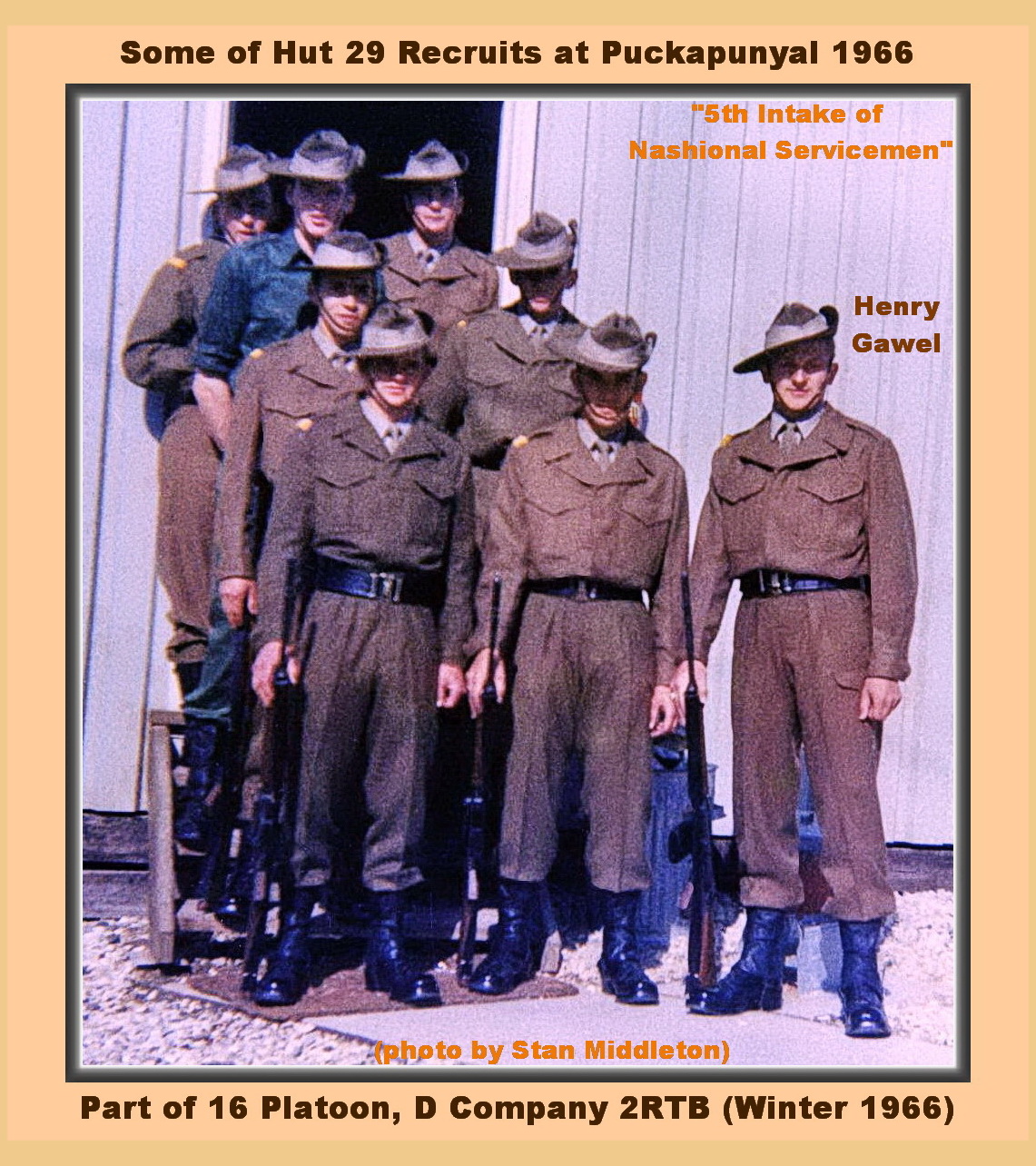The image depicts eight adult servicemen, likely Caucasian, standing outdoors against a panel wall with an open doorway. They are clad in mostly khaki uniforms, featuring black belts, black boots, and hats. However, one individual among them sports a distinctive dark blue short-sleeved collared shirt. The men hold rifles vertically, grasping them near the top while the butts rest on the ground.

Positioned in two rows, three men stand in front on gravel ground, followed by two on the steps of a small wooden staircase, with the remaining three at the doorway. Above the photograph, there's black text on the border stating, "Some of Hut 29 recruits at Puckapunyal, 1966," despite slight spelling variations in transcriptions. On the photo itself, orange text reads, "Fifth Intake of National Servicemen." A name, Henry Gawel, marks the figure on the far right, while the photographer's credit, "Photo by Stan Middleton," is also in orange at the bottom. The border below the photo includes the inscription: "Part of 16th Platoon, D Company, 2-RTB, Winter 1966."